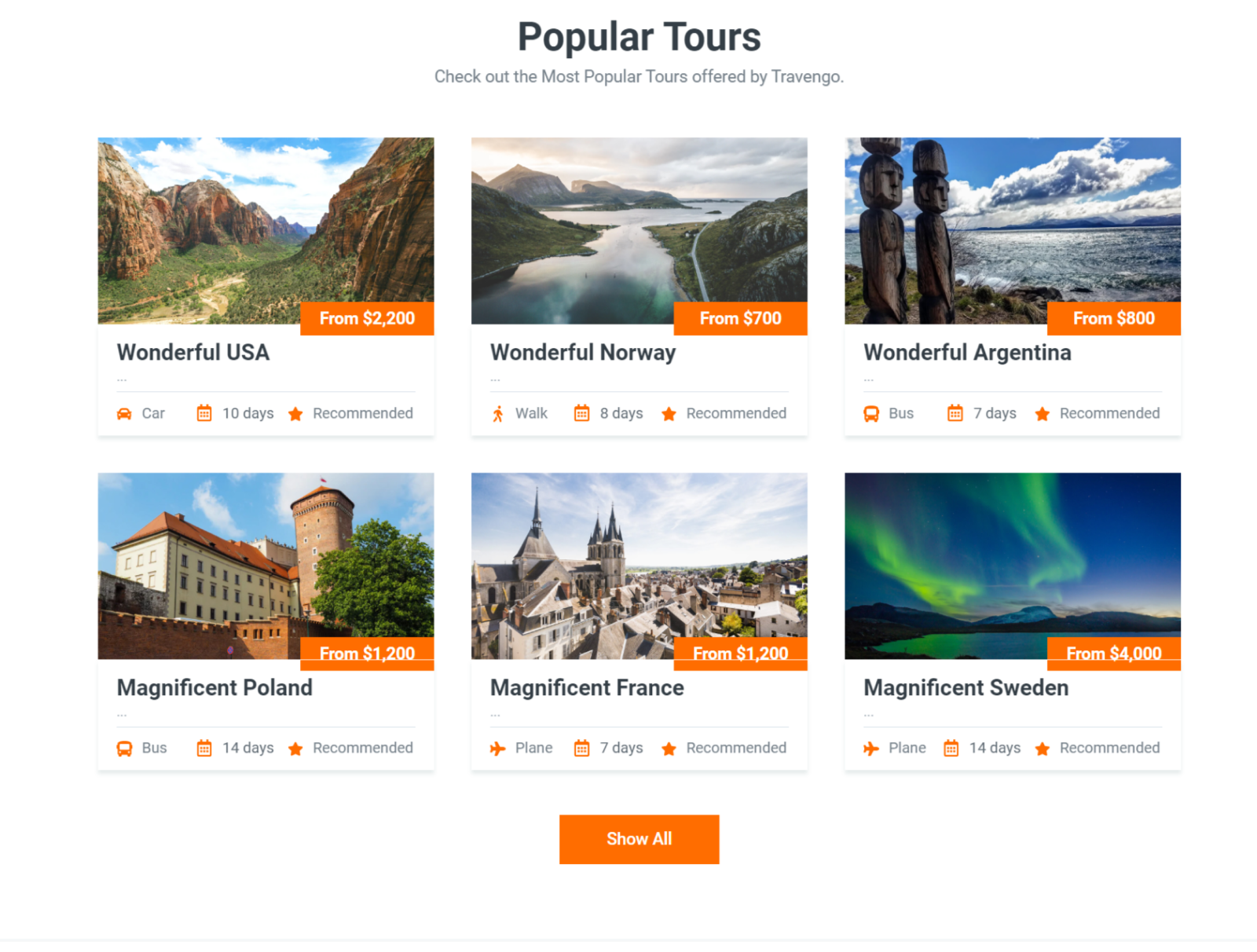Explore the most popular tours offered by Travango, all highly recommended and providing diverse experiences across various captivating destinations:

1. **Wonderful USA by Car**: Embark on a 10-day road trip across the USA for $2,200. This tour promises an immersive experience exploring iconic American sites.

2. **Wonderful Norway**: For $700, enjoy an 8-day walking tour amidst the stunning landscapes of Norway. This adventure provides an intimate connection with nature.

3. **Wonderful Argentina**: Discover Argentina on a 7-day bus tour for $800. This journey offers a blend of vibrant cities and breathtaking natural wonders.

4. **Magnificent Poland**: Explore Poland over 14 days by bus for $1,200. This extensive tour covers rich cultural heritage and picturesque landscapes.

5. **Magnificent France**: For $1,200, take a 7-day plane tour through the enchanting regions of France, from its historic landmarks to its charming countryside.

6. **Magnificent Sweden**: Experience Sweden over a luxurious 14 days by plane for $4,000. This tour offers a comprehensive exploration of Swedish culture and scenery.

Each of these tours provides a unique and immersive travel experience, meticulously curated for unforgettable memories.